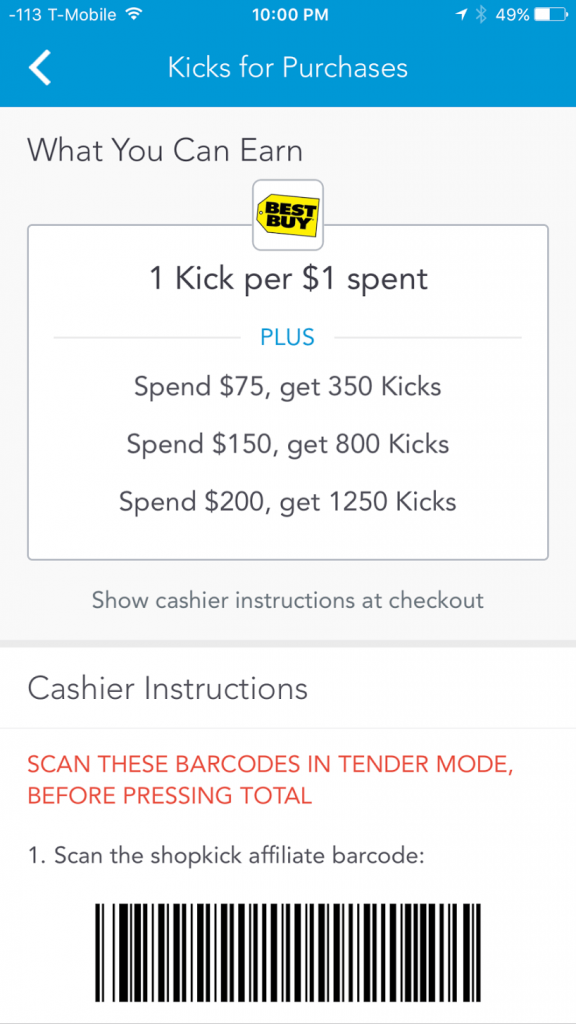The image depicts a promotional screen within a mobile application. At the top, there's a blue header with the text "Kicks for Purchases," and to the left, it displays the T-Mobile carrier information along with the time and typical phone status icons toward the right. Below the blue header, a gray section outlines the potential rewards available.

Within this gray section, it reads "What You Can Earn," followed by a box featuring the Best Buy logo. The text indicates the earning rate and various reward thresholds:
- Earn 1 kick per $1 spent, plus:
   - Spend $75, get 350 kicks.
   - Spend $150, get 800 kicks.
   - Spend $200, get 1,250 kicks.

Further instructions are provided for the cashier, highlighted in red, stating: "Show cashier instructions at checkout." Below this is a detailed procedure:
1. Scan the Shopkick affiliate barcode—the large black barcode occupies the entire bottom section of the image—in tender mode before pressing total.

Notably, the top left corner also shows "-113" next to the T-Mobile carrier name.